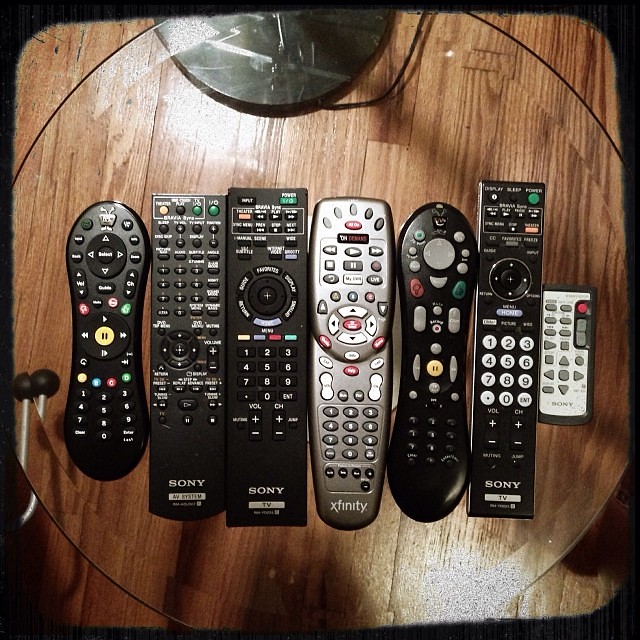This photograph captures an overhead view of seven remote controls lined up meticulously on a wooden table, allowing a clear exhibition of their varied shapes, sizes, and hues. The lineup, from left to right, starts with a rounded black remote control, followed by two rectangular black remotes, a rounded silver one, another rounded black remote with gray buttons, a rectangular black remote with circular white buttons, and a very tiny silver remote at the end. Most of the remotes are black, while two stand out with their silver or chrome appearance. The remotes appear somewhat vintage, predominantly made of plastic, and include brands such as Sony and Xfinity. Positioned on a wooden table adorned with visible wood grain, and possibly showcasing the base of a television or a lamp at the table's edge, the photograph is simple yet rich in detail, offering a glimpse into the assortment of remote controls.